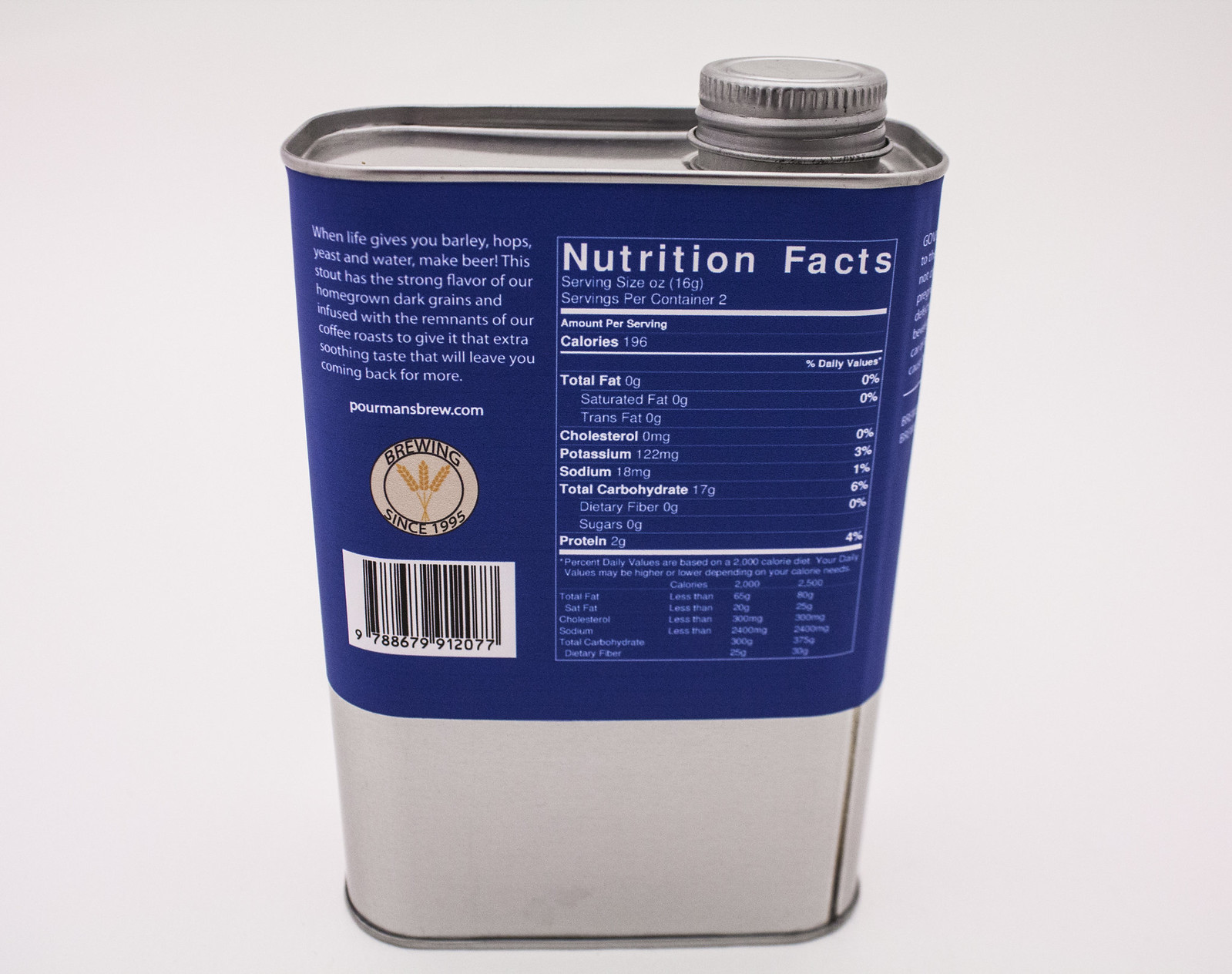The image showcases a rectangular, silver metal tin with a screw-on lid positioned on the top right. The tin is predominantly covered by a blue label that occupies the top two-thirds of the container, leaving the bottom portion exposed and reflective, almost chrome-like in appearance. The label is detailed with both text and graphics. At the top of the label, a paragraph reads: "When life gives you barley, hops, yeast, and water, make beer. This stout has the strong flavor of our homegrown dark grains and is infused with the remnants of our coffee roast to give it that extra soothing taste that will leave you coming back for more." Beneath this, the website "poormansbrew.com" is listed. A circular logo featuring yellow wheat with the words "Brewing since 1995" is also present. The back of the tin includes a barcode and a nutritional facts section detailing that the beer contains 196 calories, 3% potassium, 1% sodium, 6% total carbohydrates, 4% protein, and negligible amounts of trans fat, dietary fibers, and sugars. The can stands out against a grey backdrop, occupying approximately 75% of the image space.